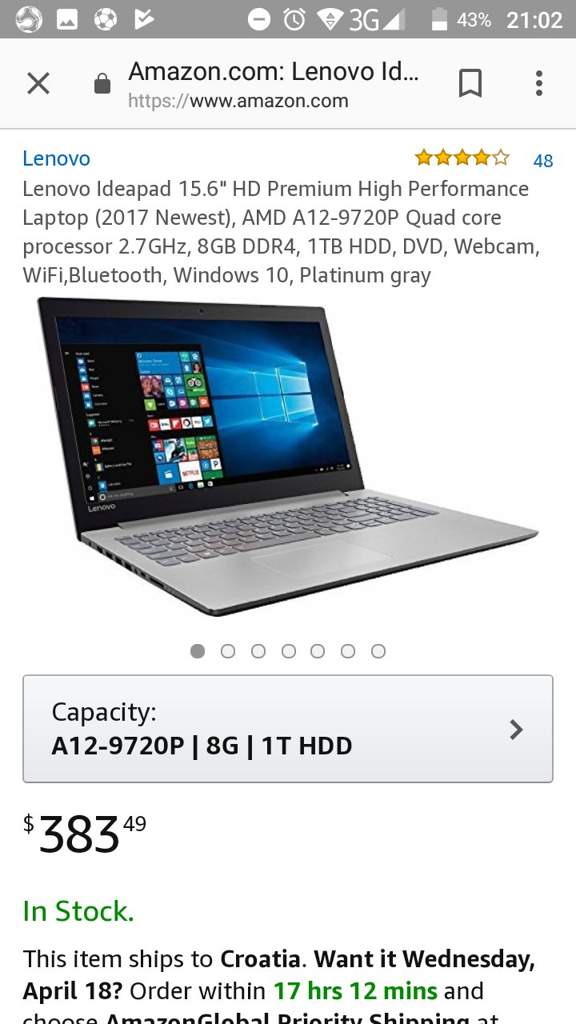This image is a detailed screenshot of the Amazon shopping website captured on a smartphone. The background is predominantly white. At the very top of the screen, there is a gray menu bar featuring an assortment of icons, including a screenshot icon, a game-related icon, a Play Store icon, a Do Not Disturb icon, an alarm, Wi-Fi, mobile network signal, battery percentage, and the current time.

Beneath this menu bar, the main content of the screenshot begins. At the very top left, there is a cross icon indicating the option to close the window. Next to it, the web address bar starts with the site name at the top, reading “amazon.com Lenovo ID”. Below, the URL is displayed as “HTTPS www.amazon.com”, followed by a bookmark icon and a three-dot menu/settings icon on the right side.

The main section of the page focuses on a product listing for a laptop. At the top left of this section, the product name is displayed: "Lenovo Ideapad 15.6 inches HD Premium High-Performance Laptop (2017 Newest)." To the right, the product rating is shown, boasting a score of 4 out of 5 stars based on at least 48 reviews.

Below the product name, there's a brief description providing specifications: "AMD A12-9720P Quad-Core Processor 2.7GHz, 8GB DDR4, 1TB HDD, DVD, Webcam, Wi-Fi, Bluetooth, Windows 10, Platinum Gray." Accompanying this description, there is an image of the laptop itself, showcasing its platinum gray color. The laptop screen visible in the image has the wallpaper and start menu icons.

Below the main image, there are dots indicating the availability of multiple images. Each dot, when clicked, displays a different perspective or detail of the product.

Further down, there is a gray button providing additional options for changing or selecting different specifications. The current specifications listed are “Capacity: A12-9720P, 8GB, 1TB HDD”.

The price of the laptop is displayed underneath this section as "$388.49." Below the price, there is a green indicator stating "In Stock." Following a short space, there is information about shipping, stating "This item ships to Croatia. Want it Wednesday, April 18th? Order within 17 hours 12 minutes." The final line of the shipping options is partially cut off, hinting at “Choose Amazon Global Priority Shipping at…”

This detailed caption encapsulates all visible elements in the screenshot, providing a thorough description of the smartphone display of the Amazon shopping webpage focusing on a Lenovo Ideapad laptop.